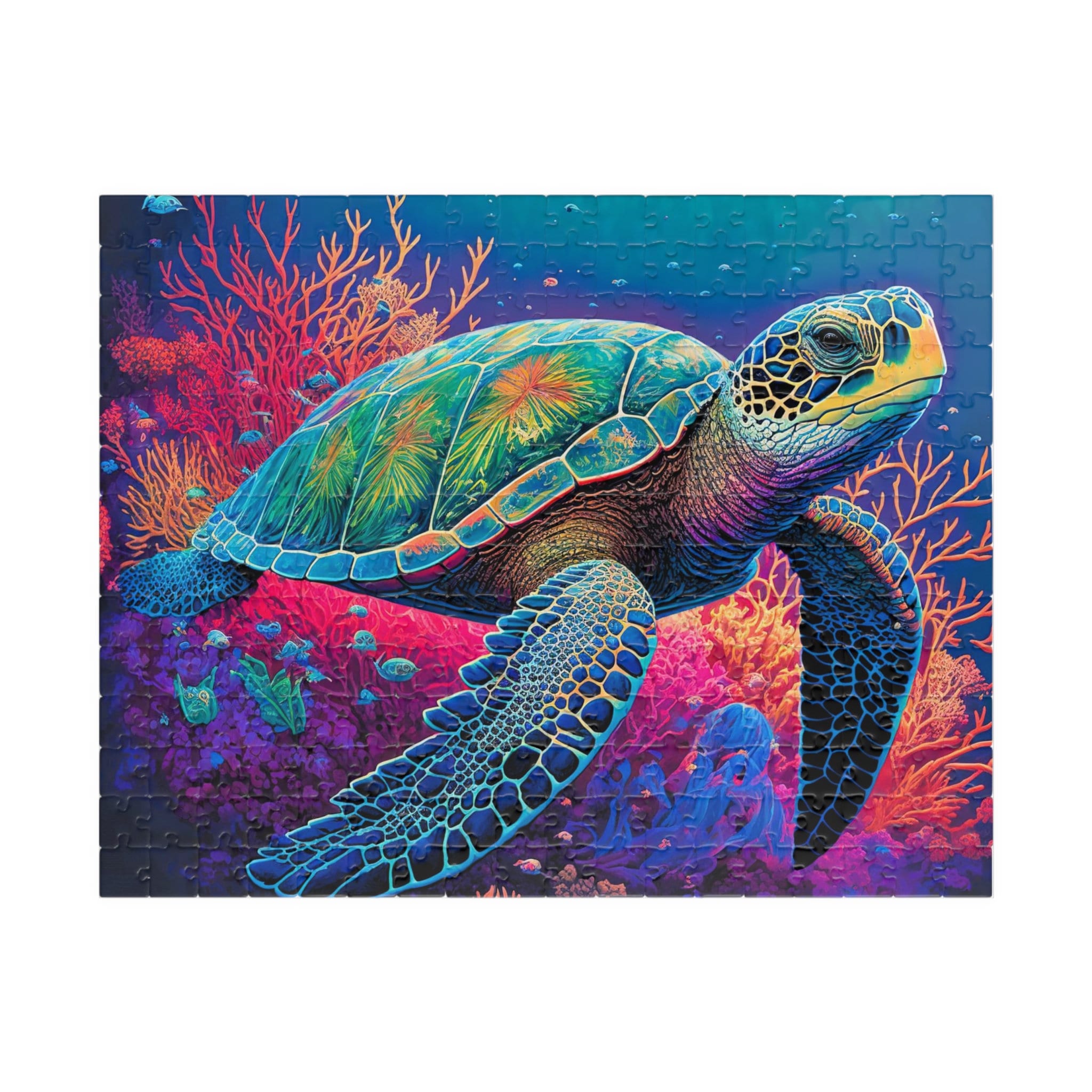This is a vibrantly colored illustration of a sea turtle swimming underwater, facing towards the right. The turtle's large shell features a mesmerizing pattern of green, blue, and orange, reminiscent of leaves or anemones. Its two front fins, blue with ridge-like textures reminiscent of rocks, are prominently visible, pointed downwards. The underside of the turtle's neck is brown transitioning to purple, and its yellow head speckled with blue boasts a visible eye looking toward the viewer.

The backdrop is a vivid blue, punctuated by colorful coral formations. On the top left side, the coral is predominantly red and orange, while orange coral extends just below the turtle's head on the right. Beneath the turtle, the seafloor is a striking pink adorned with green and blue flowers, and there appears to be green, kelp-like material. Notably, this image seems to be a photograph of a jigsaw puzzle, complete and without human presence, writing, or other animals, aside from this majestic sea turtle commanding the viewer's attention.